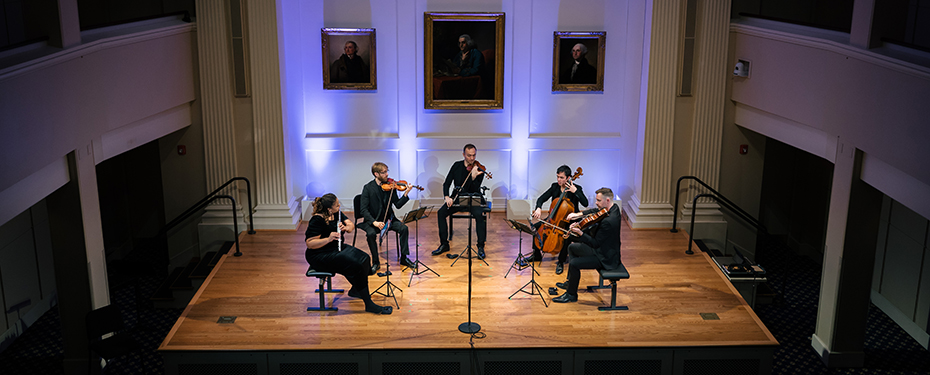The image is a color photograph in landscape orientation depicting a group of five musicians performing on a small stage in an auditorium. The musicians are arranged in a semi-circle on a hardwood floor, dressed in black outfits. From left to right, the ensemble includes a woman playing the flute, a man playing the violin, another man with a violin, a man with a bass, and another man with a large stringed instrument. Above the stage, three oil portraits hang on a white wall, each illuminated, possibly depicting the founders of the music hall. The setting includes a conductor’s stand and a microphone toward the front of the stage. Staircases on either side provide access to the stage. The photograph is taken from a higher vantage point, capturing the upper level balcony visible on both the left and right sides of the image.